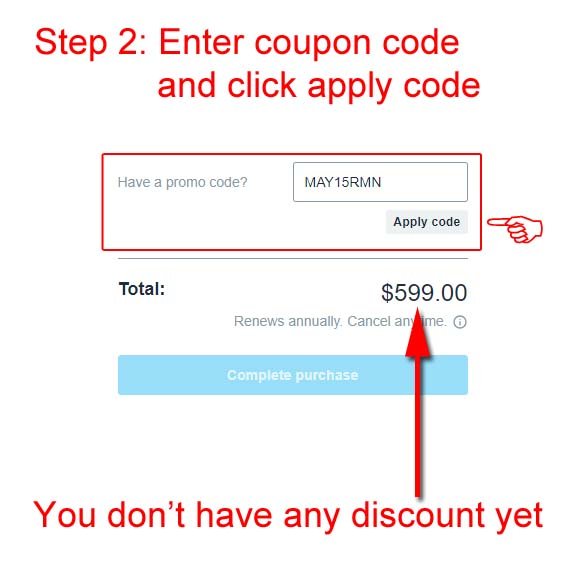The image features a white background overlaid with a combination of red, black, and blue text and graphics. At the top, prominently displayed in red text, it reads: "Step 2: Enter a Coupon Code and Click Apply Code." Below this, in black text, it asks, "Have a promo code?" providing the specific coupon code "May15RMN." 

Accompanying this input field is a button labeled "Apply Code," framed by a red outline. Adjacent to the promo code area, on the left side, a red-colored drawing depicts a hand with an extended index finger, pointing towards the promo code section.

Further down on the right, the total price is displayed boldly as "$599.00" with additional text underneath stating, "Renews annually. Cancel anytime." A red arrow, originating from the bottom right, points upwards towards the displayed price, drawing attention to the total amount.

At the bottom, a blue button with slightly dulled hues, indicating that the coupon code is invalid, is labeled "Complete Purchase." Directly beneath, in red, appears an error message reading, "You don't have any discount yet," which corresponds to the red arrow pointing to the $599.00 price, signaling that no discount has been applied.